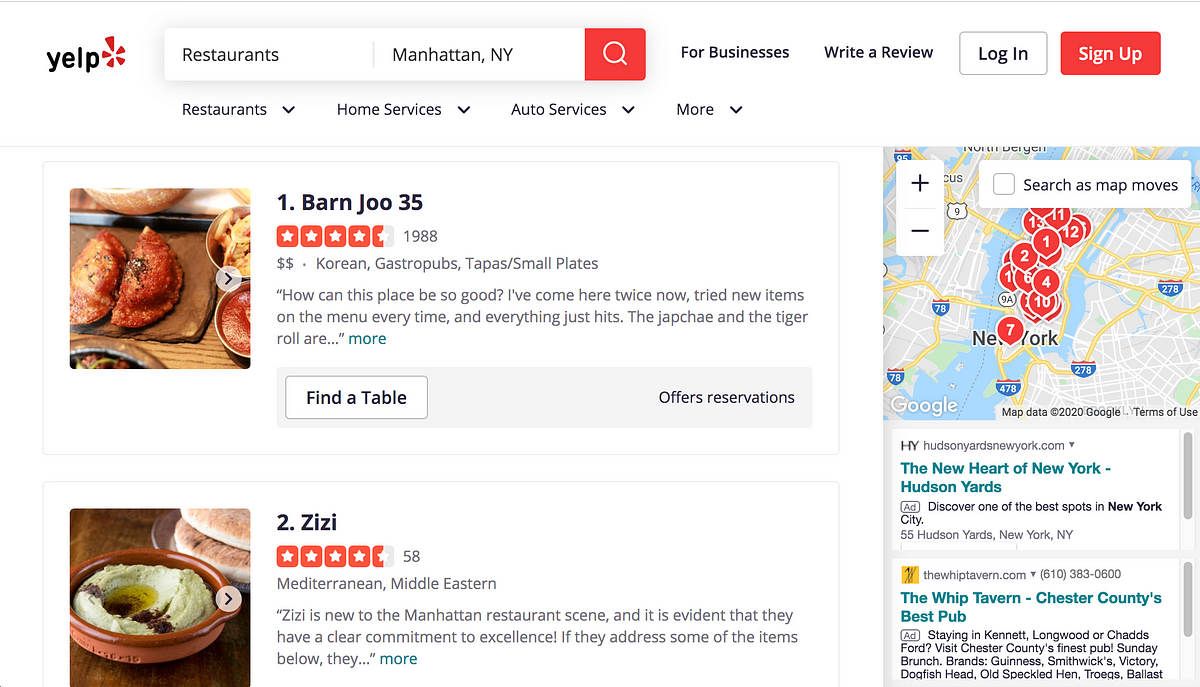The screenshot is from the Yelp website. In the upper-left corner, the Yelp logo is prominently displayed, featuring "Yelp" in black lettering alongside their iconic red logo. To its right, there is a search bar where the user has searched for "restaurants in Manhattan, New York." Adjacent to the search bar is a red square button containing a white magnifying glass. Further to the right, there are links for "Four Businesses" and "Write a Review," followed by options to "Log In" and "Sign Up."

Below these elements, a set of drop-down menus allows users to filter search results by categories such as Restaurants, Home Services, Auto Services, and more.

On the left side of the interface, search results are displayed. The first result is for "Barn Joo 35," indicating a rating, the number of reviews, and an estimated price category represented by two dollar signs. The restaurant specializes in Korean gastropubs and tapas/small plates, with a snippet of a review providing more insight. Below that, another result is listed for "ZZ’s," which offers Mediterranean and Middle Eastern cuisine.

To the right of the search results, an integrated map with red dots pinpoints the locations of the listed restaurants, enabling users to click on each dot for more detailed information.